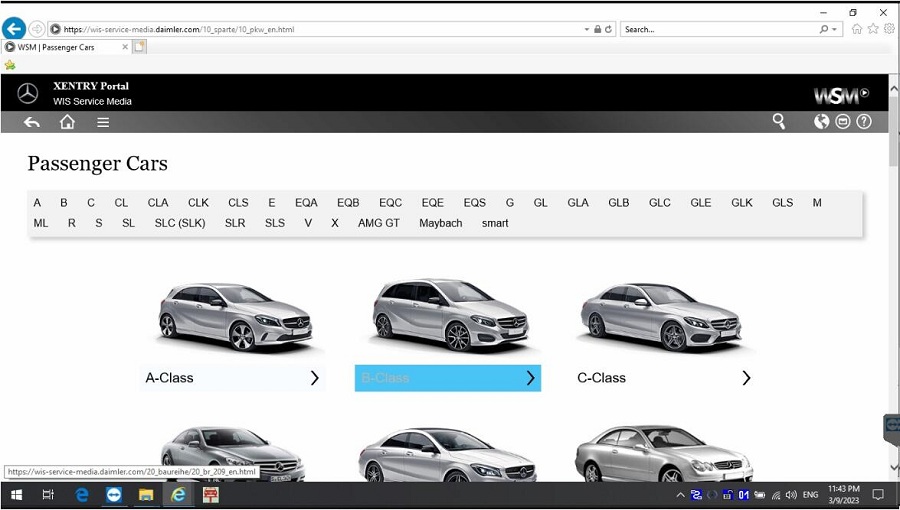Screenshot of the WSM (WIS) Cars Portal Website:

The screenshot captures a website dedicated to showcasing passenger cars from WSM (WIS). The overall design of the website features a clean aesthetic with a predominantly white background, complemented by black and gray accents. Six cars are prominently displayed, all of them passenger cars in shades of gray or silver, spanning various classes.

Visitors can easily sort through different car types using a detailed sorting section located beneath the car images. The sorting options include an extensive list of vehicle classes and models: A, B, C, C-L, C-L-A, C-L-K, C-L-S, E, E-Q-A, E-Q-B, E-Q-C, E-Q-E, E-Q-S, G, G-L, G-L-A, G-L-B, G-L-C, G-L-E, G-L-K, G-L-S, M, M-L, R-S, S-L, S-L-C (also known as S-L-K), S-L-R, S-L-S, V-X, A-M-G, G-T, Maybach, and Smart Cars.

At the top of the page, there is a sleek black bar displaying the text "X-Century Portal" and "WIS Service Media" on the left. On the right side of this bar, the WSM logo is visible, accompanied by a small play button icon. This layout and design provide a streamlined and user-friendly experience for browsing the various passenger car options available on the WSM (WIS) portal.